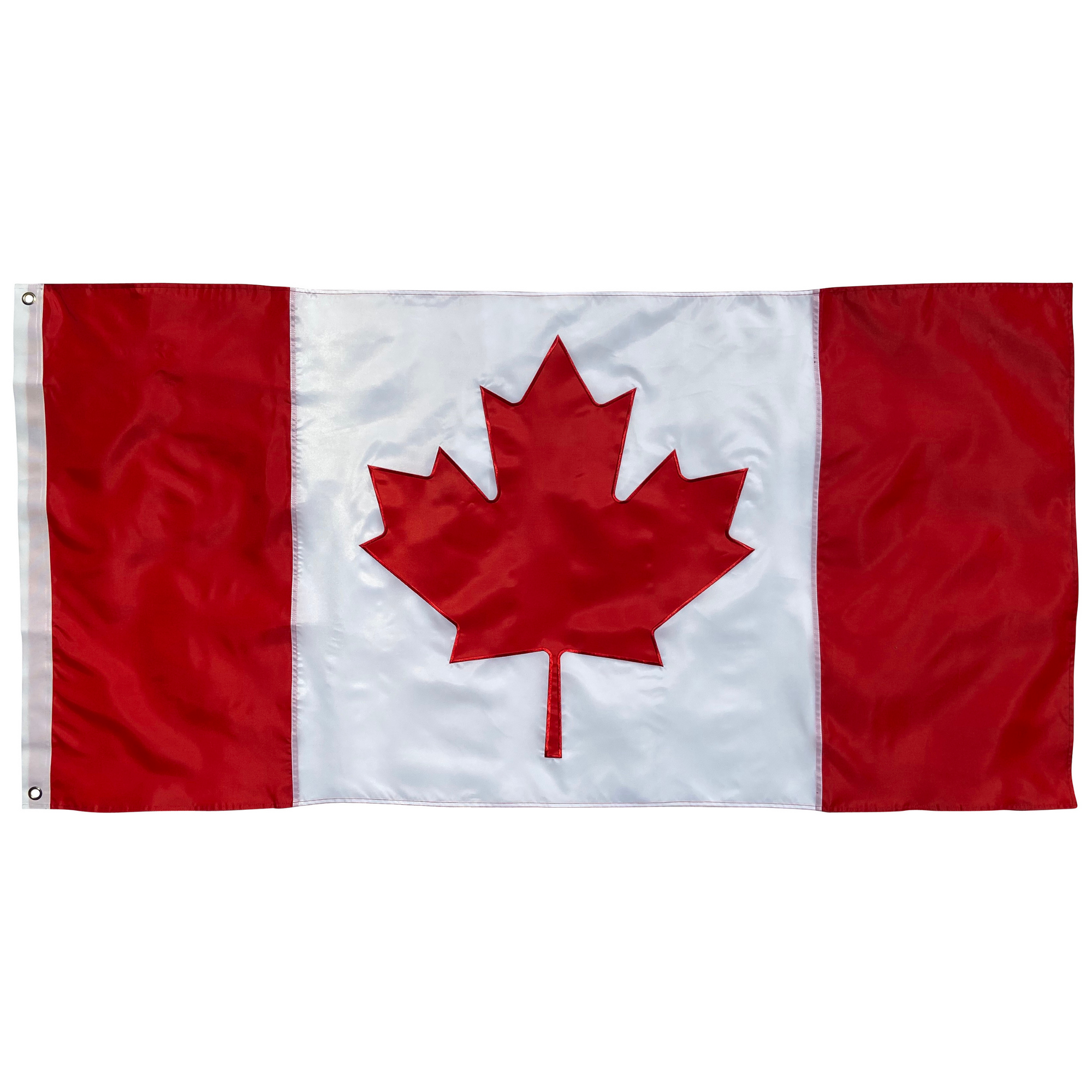This image portrays a close-up photograph of the official Canadian flag, emphasizing its prominent features. The flag consists of two vertical red stripes on either end, with a large white section in the middle, showcasing a red maple leaf at its center. The fabric appears slightly wrinkled, suggesting it is made from a durable material like cloth or vinyl, suitable for outdoor display. On the left side, there is a white strip with metal grommets for attachment to a flagpole, although it is not currently mounted. The image is tightly framed, focusing solely on the flag itself without revealing any background context, underscoring its iconic design.